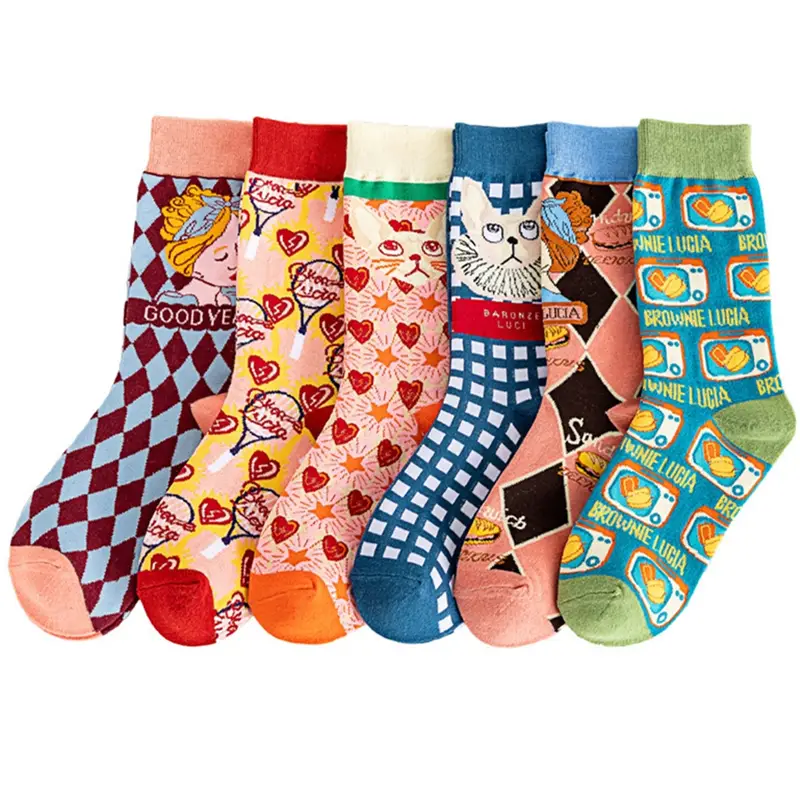This is a detailed color photograph showcasing six unique, non-matching socks, all laid out in a row against a stark white backdrop. Each sock features vibrant, fun, and funky patterns and designs. On the left, a sock with a pink toe and top displays a maroon and blue diamond-checkerboard pattern along with a cartoon princess and possibly the phrase "good year." Next, a sock adorned with red hearts and hot air balloons has an unreadable text pattern. Following that, another sock showcases red hearts and a cartoon cat among stars, complete with an orange toe detail. The fourth sock, in blue with white squares, features a cute dog looking up. Further along, a peach-colored sock presents black diamonds and a cartoon sandwich, among other images. The rightmost sock, in green, repeatedly bears the text "Brownie Lucia" in yellow, possibly accompanied by some food imagery. All the socks are adorned with whimsical, cartoonish designs, adding a colorful and playful touch to the photograph.